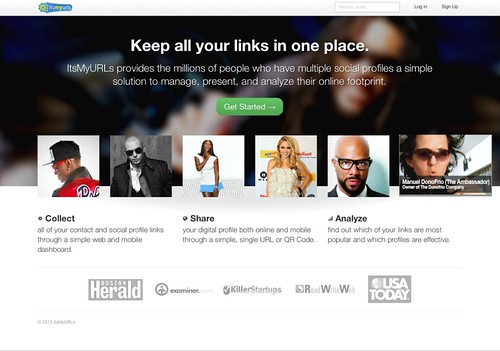The image features a prominent banner occupying most of the space. At the top of this banner, a white bar contains the company's logo on the upper left-hand corner. Despite its small size, a search bar is visible on the upper right-hand side, accompanied by login and sign-up buttons.

Beneath this white bar is a blurry black-and-white photograph anchoring the central portion of the banner. In the background of the photo, a man wearing sunglasses gazes towards the camera, though his body is angled towards the bottom left of the image. Superimposed over this image is bold, white text that reads, "Keep all your links in one place."

Below this tagline, additional text explains the product: "It's My URLs provides millions of people who have multiple social profiles a simple solution to manage, present, and analyze their online footprint." Just below this explanatory text, there is a conspicuous "Get Started" button.

Further down, the image displays six smaller pictures of musical artists. Beneath these photos, three brief blurbs are visible, each with a specific label: "Collect," "Share," and "Analyze."